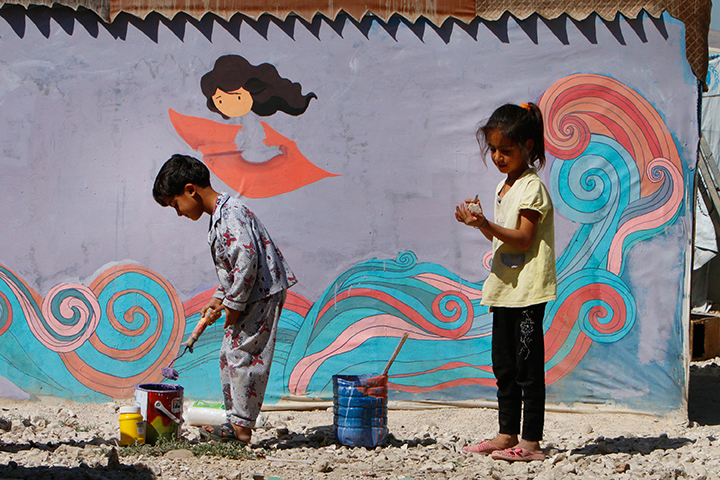In this vibrant and sunny outdoor photograph, two young children—likely around six or seven years old—are engaged in a creative activity. At the center left stands a girl with a ponytail, donning a yellow t-shirt and black pants adorned with a white flower motif. She wears pink sandals and intently holds an object in her left hand, possibly a rock, while her hand shows traces of paint. Beside her is a blue paint can with a brush inside.

Next to her is a boy dressed in gray and red pajamas with black sandals. He seems absorbed in his task as he lifts a paint roller with purple paint from a bucket, his gaze focused on the mural behind them. The mural, partially completed on a wall, showcases a series of dynamic blue, orange, and pink swirls, resembling ocean waves. Above these swirls, a cartoon woman begins to take shape, though she is still unfinished, with parts of her face, hair, and a hinted orange dress visible.

The ground they stand on is a mix of grass and a sandy texture, and additional containers, possibly a cut water jug and another paint bucket, lie nearby with various painting supplies. The children appear to be in the midst of painting this colorful mural, their youthful energy and concentration captured beautifully in the bright daylight.